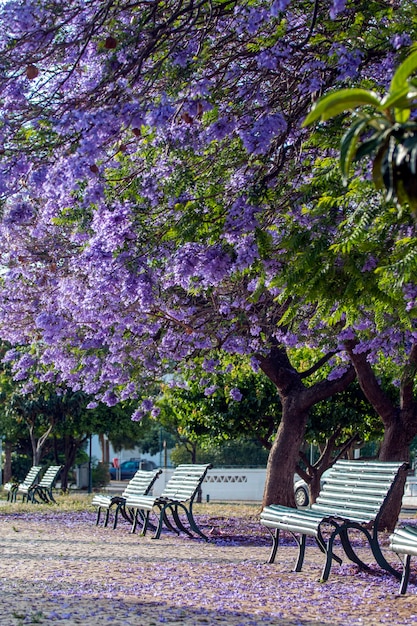This high-quality photograph captures a serene and picturesque scene in a park. The ground is scattered with vibrant purple flower petals, lending a touch of natural beauty to the setting. Several dark-colored benches are arranged throughout the area, inviting visitors to sit and enjoy the tranquility.

In the foreground, green leaves frame the image, leading the eye to a sturdy brown tree trunk adorned with a profusion of lush, purple blossoms. The flowering tree stands out magnificently, its blossoms full and vibrant. 

Beyond this tree, a backdrop of green leafy trees adds depth to the composition. In the far distance, there are faint glimpses of cars and what appears to be a white fence, hinting at the park's boundaries. Shadows dance across the flower petal-strewn ground, adding texture and contrast to the scene.

The image also captures rays of sunlight filtering through the trees, highlighting different elements and creating a dappled light effect on the petals below. Each bench and petal is crisply defined, reflecting the superior clarity and quality of the photograph.